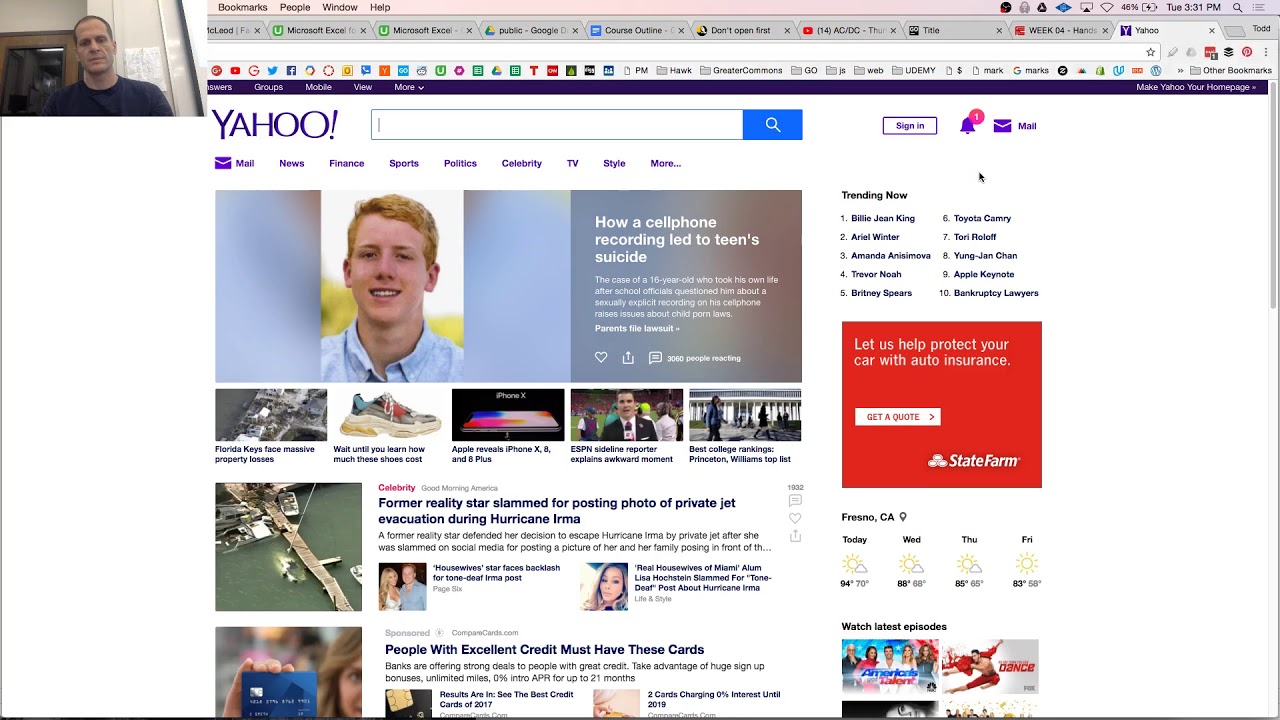A detailed screenshot captures a Yahoo homepage being screen-shared by a man in his 40s or 50s with a receding hairline and short hair, seated in what appears to be an office. The man, wearing a gray t-shirt, faces the camera directly. Behind him, a brown door with a window leading to another room with white walls can be seen. The browser displays multiple tabs, about seven or eight, but the focus is on the Yahoo tab. The toolbar appears cluttered with numerous icons.

The Yahoo homepage prominently features the purple Yahoo logo with an exclamation point, a search bar, and options to sign in, along with a notification and a mail icon. The main news story discusses a cell phone recording that led to a teen's suicide, showing an image of a young boy with white skin, red hair, and a blue collared shirt. An advertisement for State Farm in red with white lettering is positioned to the right. The location is marked as Fresno, CA, displaying the weather icon. Additional news stories and ads populate the lower part of the page.